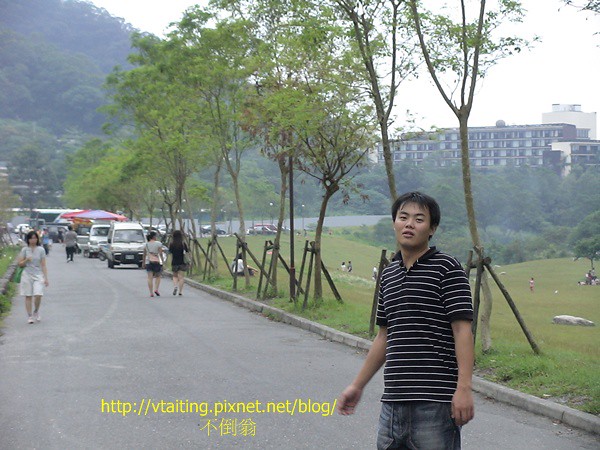In this detailed photograph, an Asian gentleman stands on a grey-colored street, looking directly at the camera. He is dressed in a black t-shirt adorned with white lines and wears blue jeans. The scene around him is bustling and vivid; behind him, other people can be seen walking along the street, framed by parked vehicles.

To the right of the street, there is an uneven grassy ground where a few more individuals are seated and umbrellas are visible. In the distance, a hill lush with trees rises, with buildings—including what appears to be a large hotel—nestled on its right side.

The environment is further enriched with trees lining the road and an impression of a parkway. Red and grey tents, possibly set up for an event, are also seen in the background along with a large apartment building in the far distance. The bottom middle of the image features text in yellow, reading "http://vtaiting.pixnet.net" along with some Chinese characters.